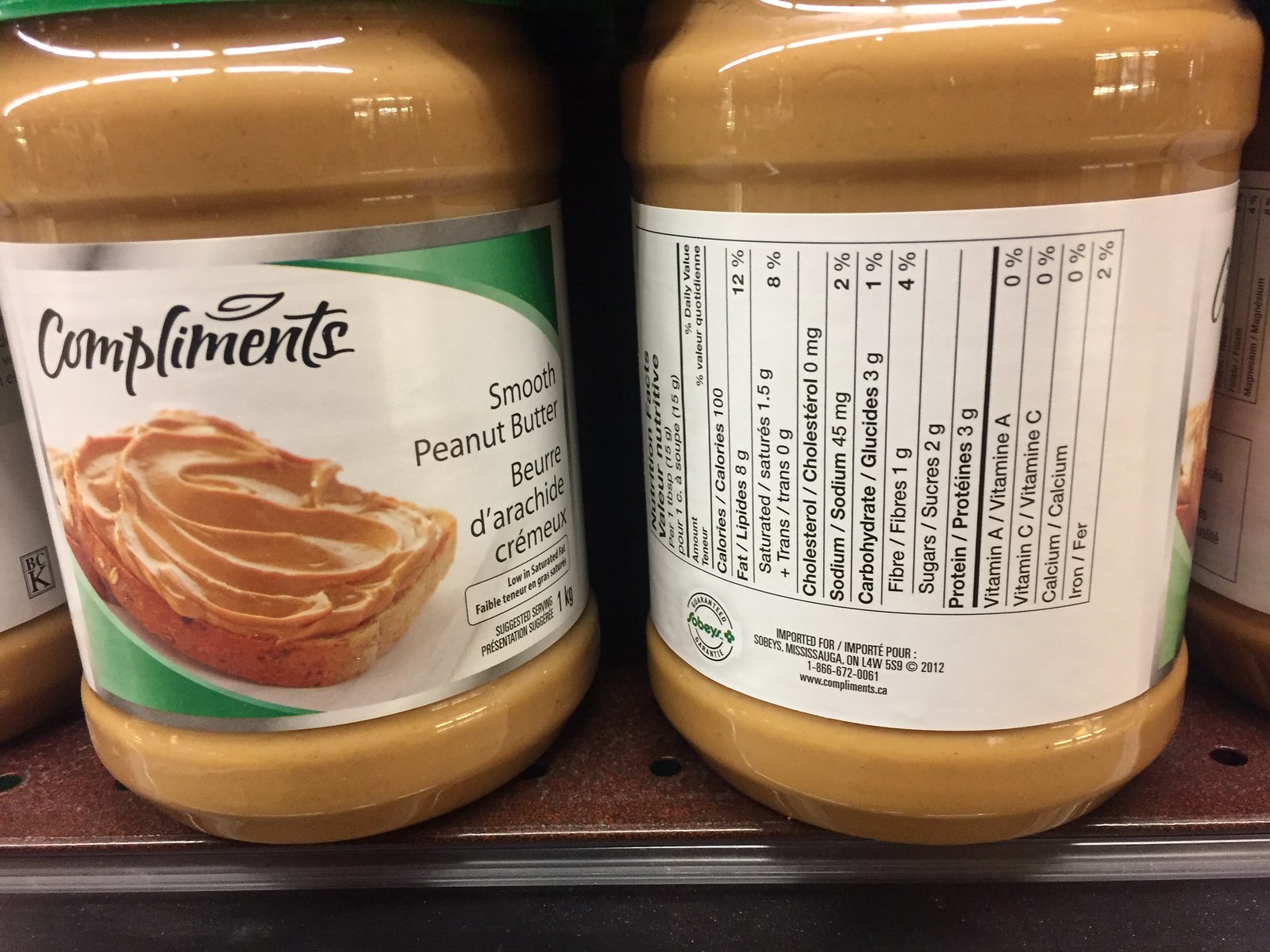The image depicts two clear plastic jars of Compliments Smooth Peanut Butter sitting on a store shelf. The jar on the left prominently displays the front label. This label features a silver frame and a white background with green accents in the top right and bottom left corners. The brand name "Compliments" is written in black lettering above a piece of wheat toast with peanut butter spread on it. Below this, in black lettering, it states "Smooth Peanut Butter," followed by its French translation, "Beurre d'Ariche Crèmeux." The jar on the right shows the back of the label, displaying nutritional facts and ingredients, such as calories (100 per serving), fat content (12%), saturated fat (8%), zero cholesterol, sodium (2%), carbs (1%), and fiber (4%). Both jars allow visibility of the light brown peanut butter inside. The shelf they rest on has a gray front and black top, featuring small holes along its edge.